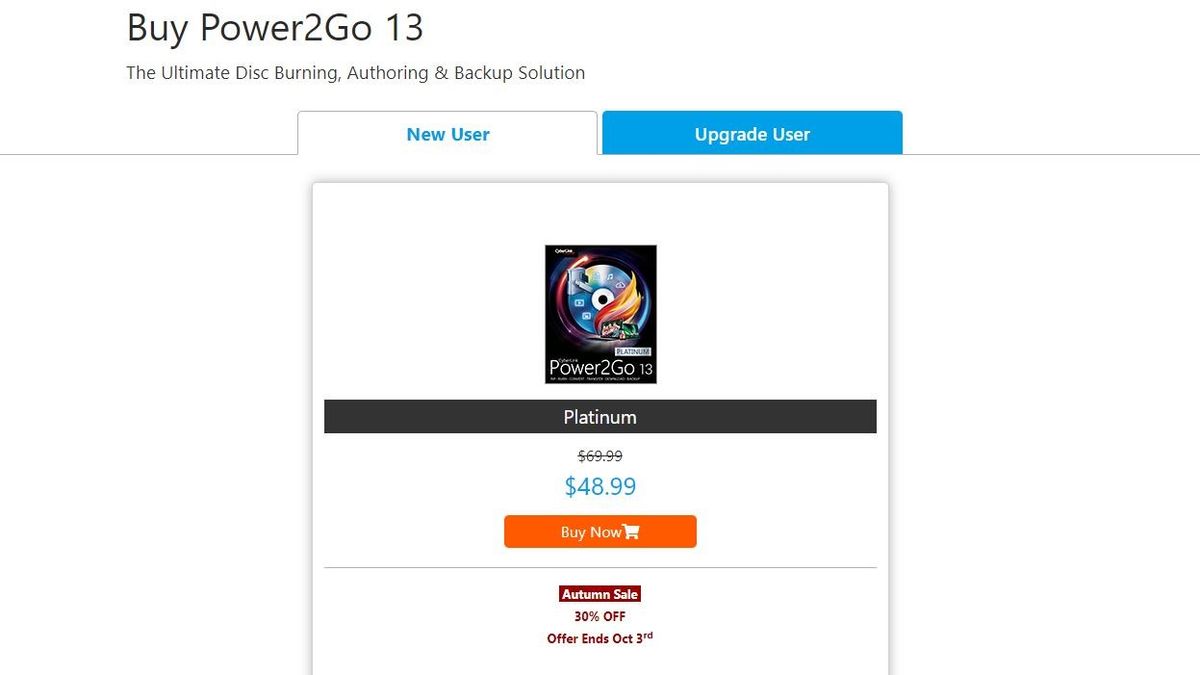In the top-left corner of the image, the text reads "Buy Power2Go 13: The Ultimate Disk Burning, Authoring, and Backup Solution." A grey line runs horizontally, then vertically upwards, horizontally again, downwards, and finally resumes its horizontal course. Where the line ascends, "New User" is written in blue, and beside it, a blue rectangular tab labeled "Upgrade User" is displayed. Below this, there's a partially outlined white box, marked in grey on three sides, featuring a small logo resembling a clock with flames or hair. The text in this section states "Power2Go 13."

Beneath this box, a black rectangle displays "Platinum" and lists the price as $69.99, which is crossed out. Below the original price, in blue, the discounted price of $48.99 is shown. Adjacent to this, an orange rectangle contains a "Buy Now" button alongside a shopping cart icon. Further down, a thin grey line separates this section from a red rectangle announcing an "Autumn Sale - 30% Off" in white text. Directly below, in red text, it reiterates "30% off, Offer ends October 3rd."